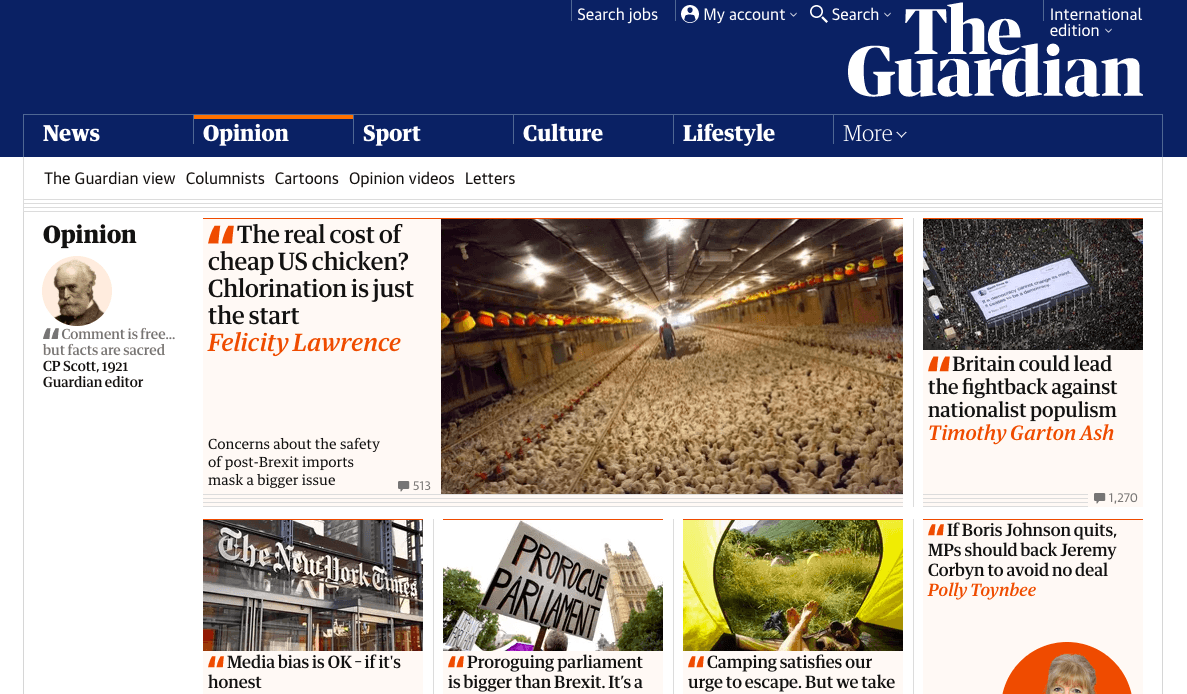Here is a cleaned-up and detailed caption:

---

This screenshot captures a webpage from The Guardian, showcasing its international edition. The page header features a blue background with options for "Search Jobs," "My Account," and "Search," listed on the right side. Along the top navigation bar, various sections like News, Opinion, Sport, Culture, Lifestyle, and more are outlined from left to right. Beneath this navigation bar, there are further categories including "The Guardian View," "Columnists," "Cartoons," "Opinion," "Videos," and "Letters."

Highlighted prominently on the page is a quote from CP Scott, a Guardian editor from 1921, stating, "Comment is free, but facts are sacred." 

On the right, several opinion pieces and quotes are displayed, including "The real cost of cheap US chicken: Coronation is just the start" by Felicity Lawrence, discussing concerns about the safety of post-Brexit imports in light of broader issues. Another quote reads, "Britain could lead the fight back against nationalist populism" by Timothy Garton Ash.

Below these sections on the left side, there is an image of the New York Times building with a headline discussing media bias: "Media bias is okay if it's honest." Adjacent to it, a photo of a protest sign reads, "Proroguing Parliament is bigger than Brexit." Nearby, another image conveys the sufficiency of camping in fulfilling the desire to escape daily life. Lastly, another headline by Polly Toynbee opines, "If Boris Johnson quits, MPs should back Jeremy Corbyn to avoid a no-deal Brexit."

---

This detailed caption provides a comprehensive overview of the content and layout of the webpage captured in the screenshot.